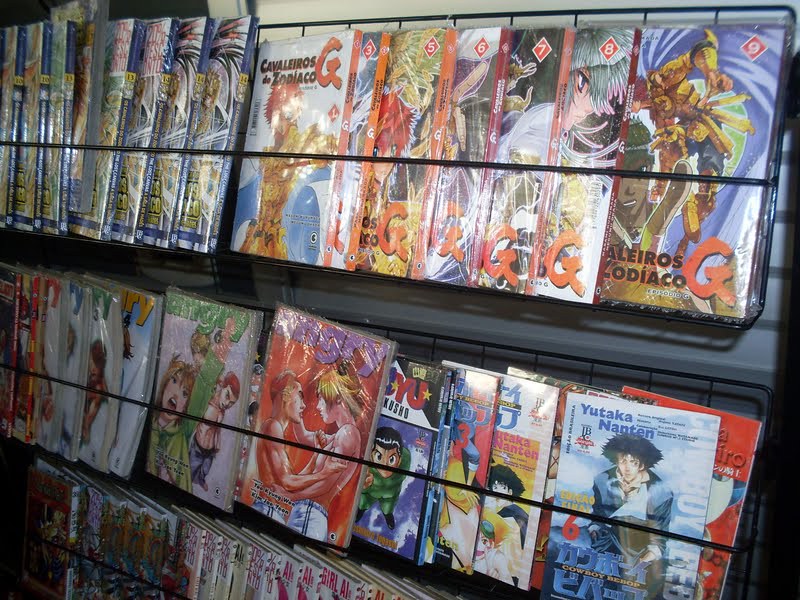This full-color indoor photograph captures a display of comic books or magazines on a wire rack against a white wall. The rack features three rows, each densely packed with anime-themed comics or games, identifiable by their distinctive artwork and titles. While most titles are unreadable due to the distance and angle of the photograph, the top row includes items shrink-wrapped in plastic, such as "Cavaleros de Zodiaco" and another with a prominent orange "G" on the spine. On the far right, a title numbered nine in a series is visible, and below it, additional shrink-wrapped items obscure cover details due to reflection. The bottom row features "Yutaka Nanten," highlighted by an illustration of a dark-haired man. The overall theme appears to focus on traditional young-adult anime adventures, rather than space, monsters, or humor.